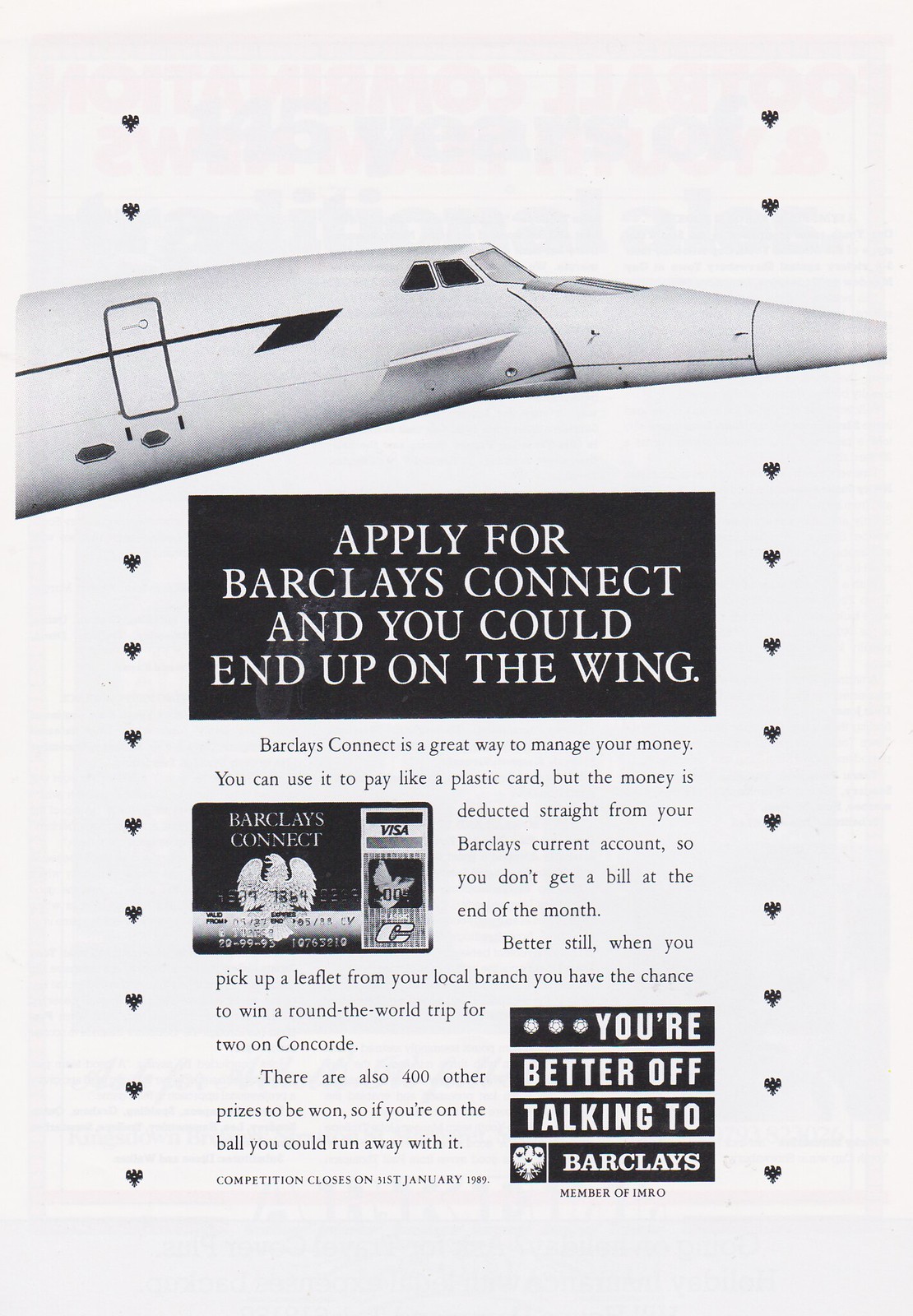Set against a white background with heart-shaped black borders on either side, the image features a notable black and white illustration of an airplane's nose and windows at the top. Below this, a prominent black box with white text reads, "Apply for Barclays Connect and you could end up on the wing." Underneath, in paragraph form on a white background with black text, the promotion details that "Barclays Connect is a great way to manage your money. You can use it like a plastic card, but funds are deducted directly from your Barclays current account, eliminating any end-of-month bills." The text further entices readers by highlighting an opportunity: "When you pick up a leaflet from your local branch, you could win a round-the-world trip for two on Concord, along with 400 other prizes. The competition closes on January 31st, 1989." At the bottom, the tagline, "You're better off talking to Barclays," encourages engagement. An image of a Barclays credit card complements the text, enhancing the promotional message.